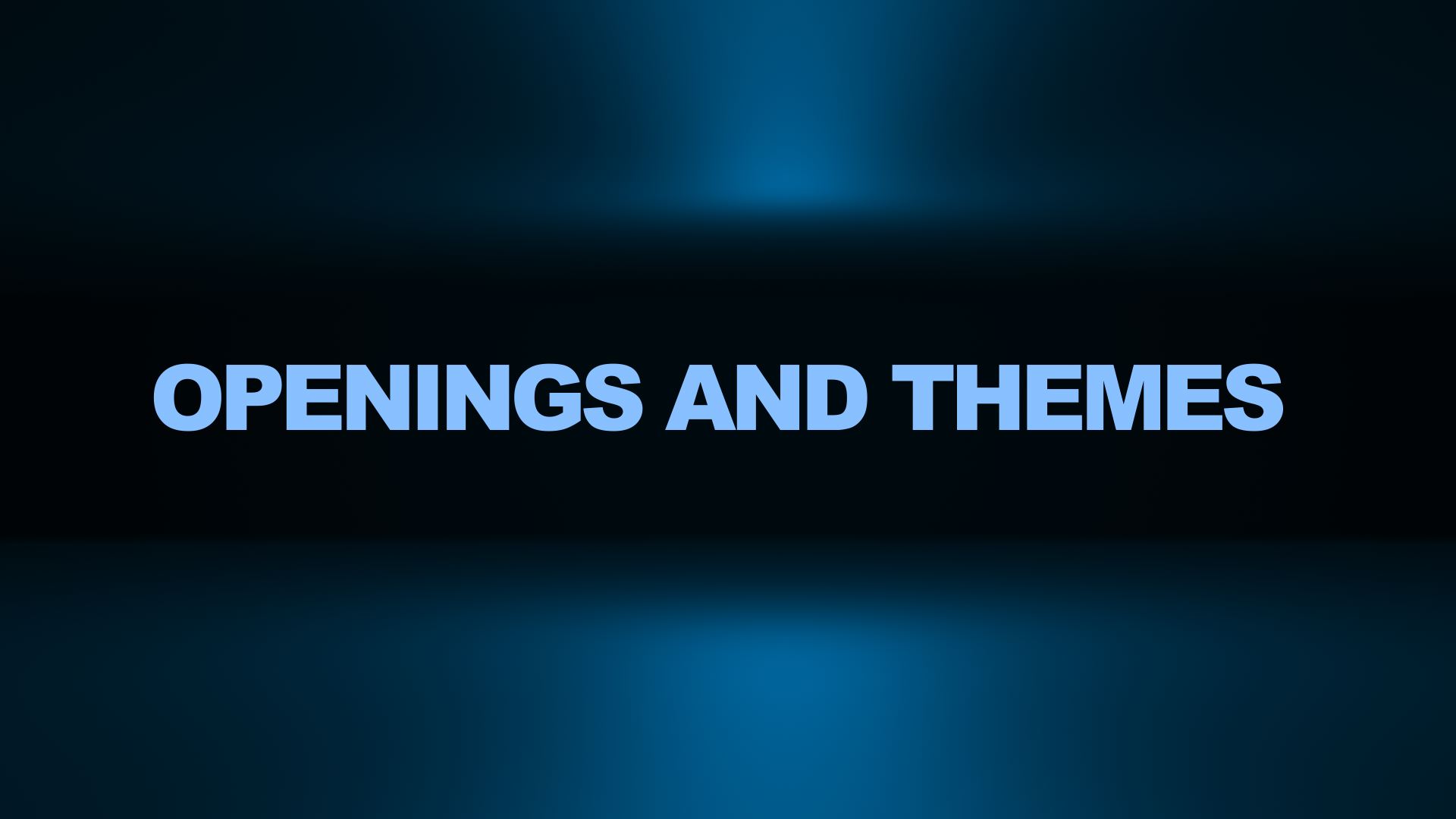The image displays a rectangular slide with a gradient blue background that transitions from dark blue in the corners to a lighter blue, almost white, near the center. The middle of the slide features the phrase "OPENINGS AND THEMES" in all capital letters, rendered in a light sky blue color that contrasts starkly against the darker central background. This central area is nearly black, creating an ombre effect that enhances the legibility of the text. There are no additional graphics or artwork, suggesting this is likely the introductory slide of a presentation, poised to outline the themes to be discussed, but without any further contextual clues about the subject matter.